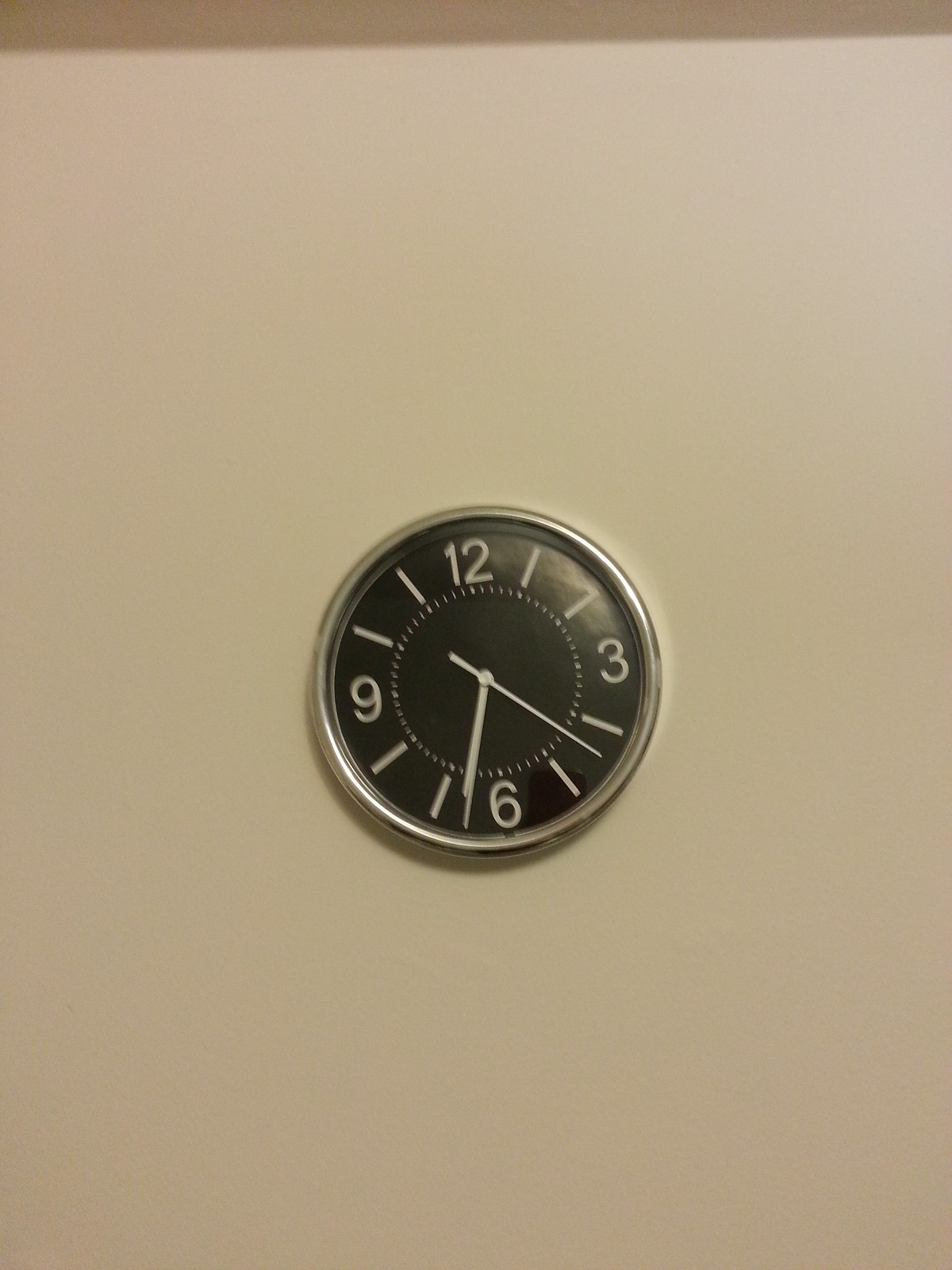This detailed photograph captures a large, circular clock mounted on a plain white wall, with a slightly darker shadow casting over the top of the wall and visible beige ceiling. The clock itself features a sleek black face with prominent white numbers at the 12, 3, 6, and 9 positions. Each of the remaining hours is marked by simple slashes radiating outward from the center. A silver casing encircles the clock, which also has a glass cover that reflects light at the top right corner. The clock displays the time as approximately 6:33, with the second hand positioned around the 22-second mark. This straightforward yet stylish timepiece is complemented by long, thin silver hands.